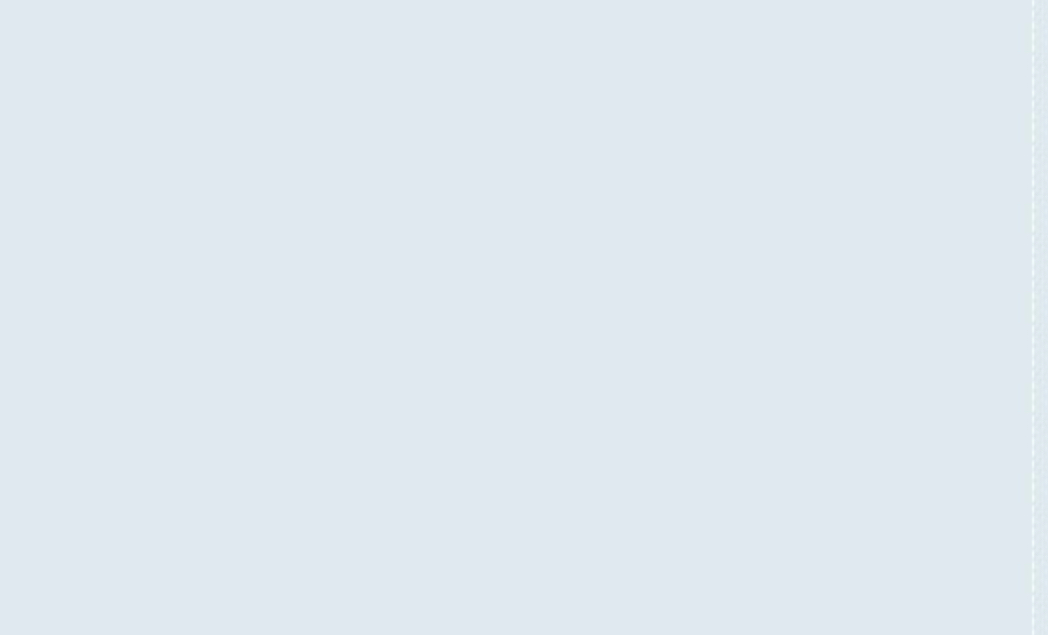This image prominently features a medium blue-gray background, reminiscent of the typical gray seen on computer screens but infused with a subtle hint of blue, giving it a slightly lighter appearance. The rectangular canvas is wider than it is tall, occupying approximately 30% to 50% of the viewing area, though the specific dimensions may vary. Notably minimalistic, the image does not present any text or central figures, maintaining a serene, unembellished expanse of color. A singular feature breaks the uniformity: a vertical, off-white, dotted line runs from the top to the bottom, situated roughly 3% in from the right edge, subtly disrupting the continuous blue-gray field. This delicate vertical accent adds just a touch of structural interest to the otherwise plain yet calming image.